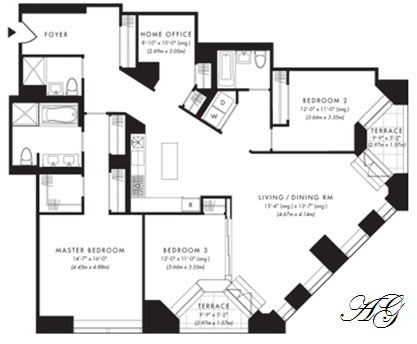A detailed black and white drawing of a house floor plan is depicted from an aerial perspective, utilizing squares and images to symbolically represent different areas. The house overall has a nearly square shape but with one corner cut off, possibly indicating the entrance. The layout prominently features an open-plan living, dining, and kitchen area.

Extending from this main area:
- Bedroom 2 and Bedroom 3 are situated adjacent to each other.
- There is a terrace, followed by another terrace that might function as a patio space.
- A washroom and a bathroom are also included.
- A home office is conveniently placed within the layout.
- The foyer, which doubles as the main entrance, is located on the opposite side of the cut-off corner.

Additionally, the master bedroom is accessible from the foyer area, leading to a walk-in closet and an ensuite bathroom. Various storage areas are dispersed throughout the plan, denoted by black segments, which could also symbolize windows, though this is unclear.

Noteworthy alphanumeric dimensions accompany the rooms, although the image is too small to read them clearly. In the corner of the drawing, the name "Adrian" is elegantly inscribed, likely indicating the architect or the designer of the floor plan.